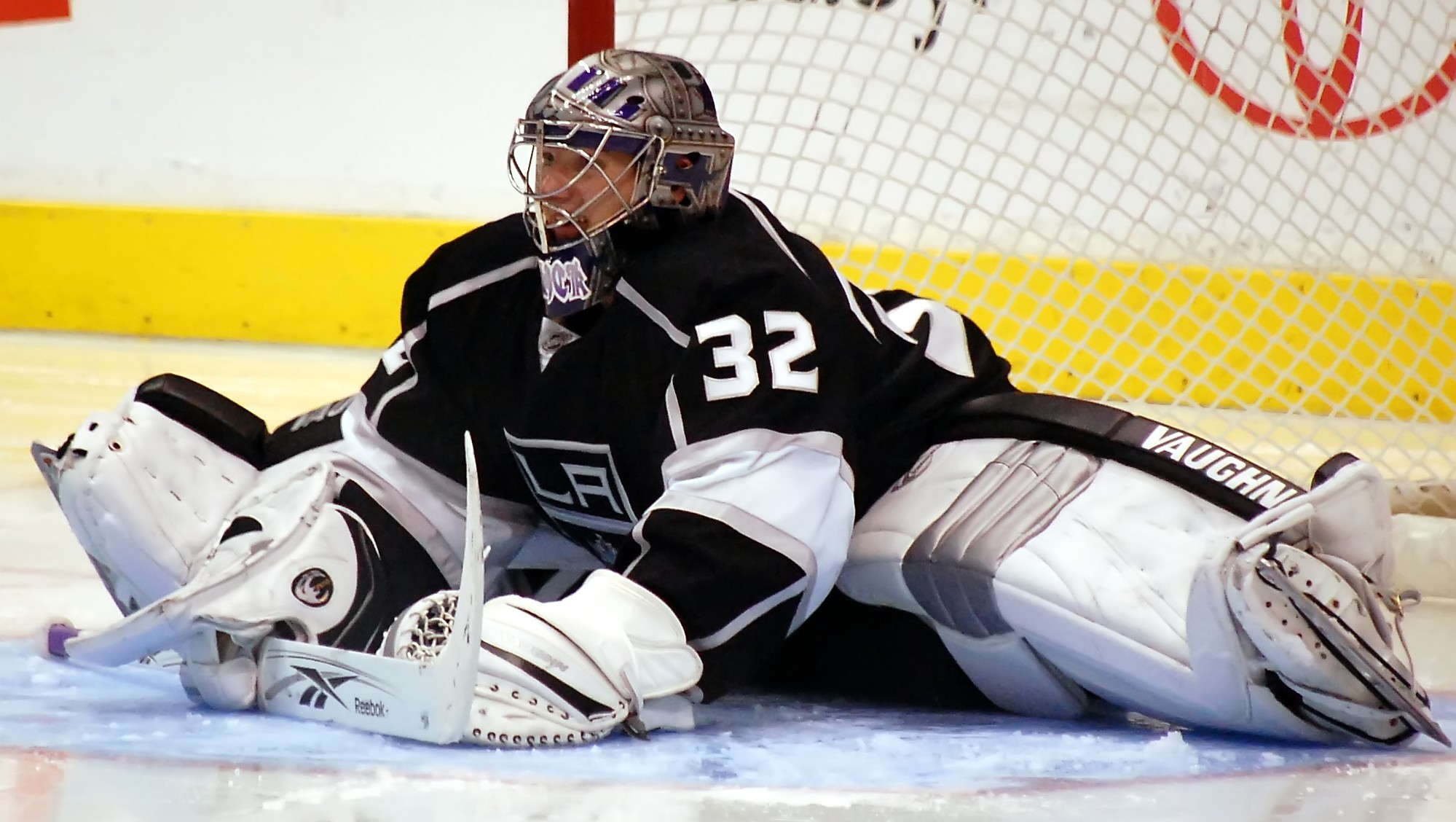In this detailed photograph, a hockey goalie identified by the number 32, in a black and white uniform with "LA" on the front, is positioned directly in front of the red-framed net. The goalie, who wears a black jersey with white sleeves, is captured performing an impressive split on the white ice. This action reveals his dedication to the game. His equipment includes a gray helmet with a cage front, large padded knee and leg protectors branded with "Vaughn," and a protective glove. The scene also features his hockey stick laying across his arms and ice skates securely on his feet. Behind him, a yellow barrier and white fencing mark the boundary of the rink, offering additional context to his surroundings.